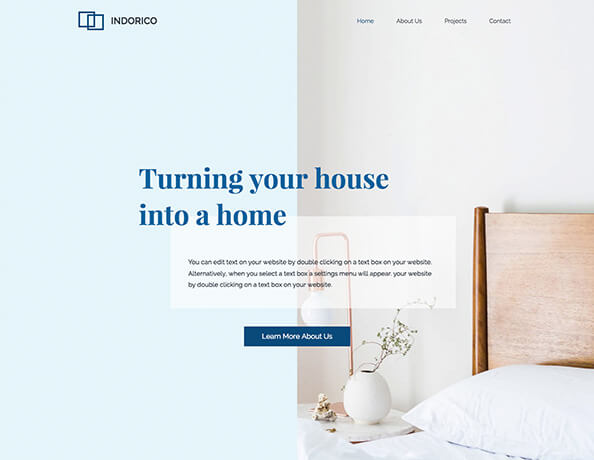The image appears to be an advertisement for a company called Indorico. The left side of the image features a light blue background with the company name "Indorico" prominently displayed at the top. The tagline "Turning Your House into a Home" is written in bold blue lettering in the center of the left side without a text box behind it. Below it, a white text box contains an instructional placeholder text about editing the website, which reads, "We can edit text on your website by double-clicking on a text box on your website. Alternatively, you can select a text box and settings menu will appear at your website."

On the right side of the image, the background is a soft off-white gray, showcasing the upper left-hand corner of a cozy bedroom. The bed features a brown headboard, white pillows, and matching white sheets and blankets. A round end table stands next to the bed, displaying a beehive-shaped vase with some greenery and a gold or copper lamp with a swooping design and a round bulb. Additionally, there is a decorative white-gray marble knickknack on the table. The top of the right side includes navigation options: Home, About Us, Projects, and Contact. At the bottom of the image, a blue box with white lettering invites viewers to "Learn More About Us."

Overall, the image blends a serene visual aesthetic with practical text elements, effectively communicating Indorico's mission to transform living spaces.